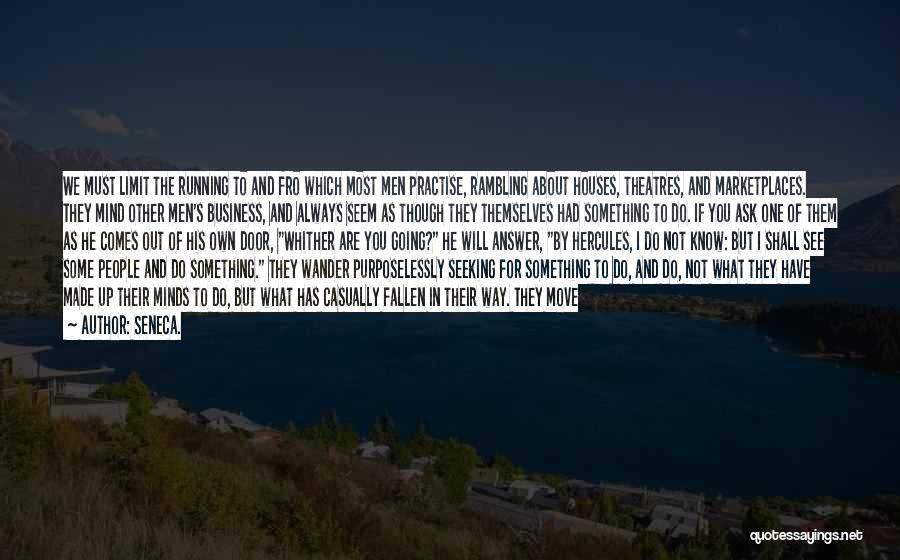The image is a darkened landscape that is difficult to make out but reveals several key features: a large lake at its center, surrounded by green grass and gray stones in the foreground. In the background, there are more details visible, including houses, trees, gardens, and white-colored buildings situated on what appears to be a hillside or mountainous area. Above, the sky is vividly blue with some white clouds. Superimposed on this dimly lit scenery is a white block of text with an inspirational quote by Seneca. The quote reads: "We must limit the running to and fro which most men practice, rambling about houses, theaters, and marketplaces. They mind other men's business, and always seem as though they themselves had something to do. If you ask one of them as he comes out of his own door, 'Whither are you going?' he will answer, 'By Hercules, I do not know, but I shall see some people and do something.' They wander purposelessly, seeking for something to do, and do not what they have made up their minds to do, but what has casually fallen in their way. They move." The quote is credited to Seneca, and at the bottom right of the image, there is a small text reading "quotes sayings dot net."